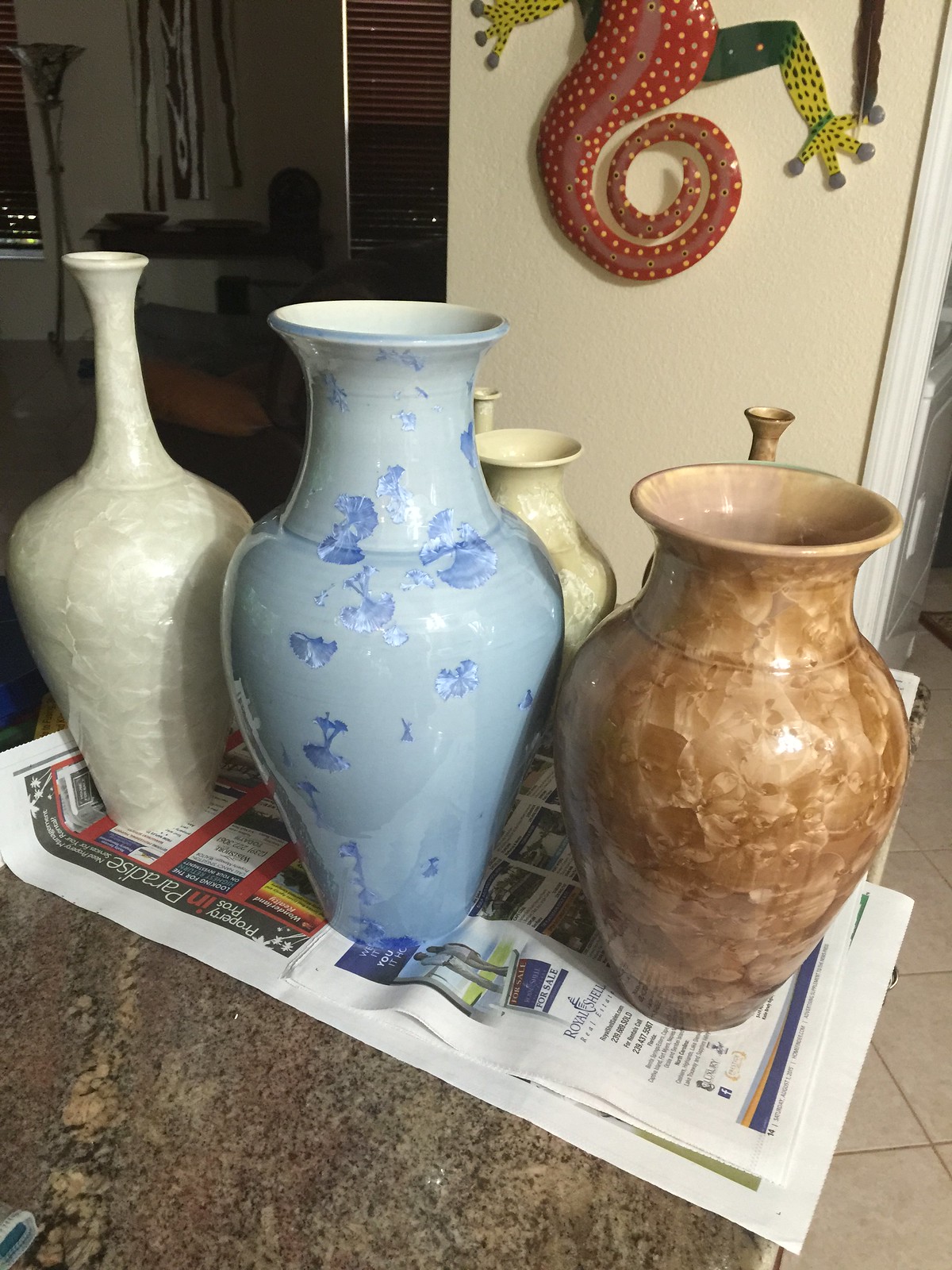This image, set in a kitchen, shows an array of ceramic vases displayed on a brown marble countertop adorned with light brown, tan, and black speckles. The vases rest on a piece of newspaper featuring advertisements. The countertop surface has a predominantly brown hue with swirling patterns of grey, mauve, and beige. 

In the foreground, the first vase to the left is a tall, slender, white vase with a long, narrow neck and a rolled top. To its right stands a larger, light blue vase adorned with dark blue floral and butterfly patterns, wider at the bottom and tapering into a cylindrical bowl with a white interior. Next is a shorter, chocolate brown vase with a textured, decoupage-like surface in various shades of brown and beige and a cream-colored interior. Partially hidden behind this vase is a small olive green one with white accents and a white interior. 

In the background, the tops of two additional vases are visible – one with a thin neck and fluted top, and another long white stem-like vase. 

Decorating the tan wall with white trim behind the vases is a colorful metal lizard, its cream-colored body transitioning to green feet with black spots, a dark green midsection, and a red tail with white spots, divided by an acrylic white line. The room features tiled brown flooring with brown grout, a window with brown blinds on the left, shelves, and a silver lampshade visible atop the counter with assorted kitchen items nearby.